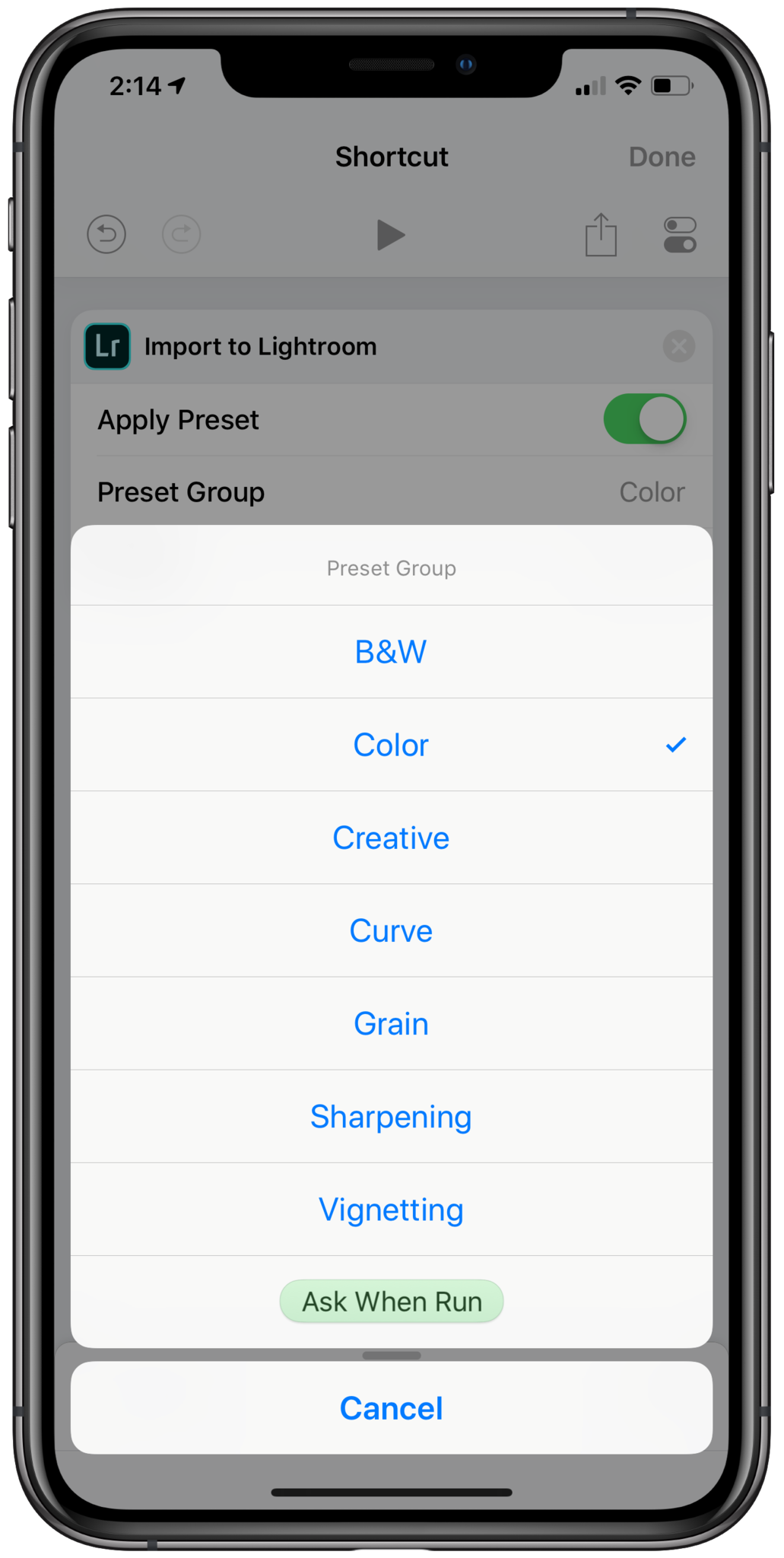The image features a smartphone with its screen clearly visible. The outer border of the phone is also shown. In detail:

- **Top Left:** The time is displayed as "2:14" next to a GPS icon.
- **Top Center:** There's a small circular cutout for the front-facing camera.
- **Top Right:** Three icons are visible — a battery icon, followed by a Wi-Fi icon, and a cellular signal icon.
  
At the mid-section of the screen:
- **Middle Left:** The word "Shortcut" is displayed.
- **Middle Right:** The word "Done" appears.

The central part of the screen has a vertical list of tabs with different options, indicating a settings or editing menu:
- "Preset Group B&W"
- "Color" (highlighted with a blue checkmark)
- "Creative"
- "Curve"
- "Grain"
- "Sharpening"
- "Vignetting"
- "Run"
- At the bottom of this list, "Cancel" is shown.

Above this section, "Import To" is mentioned, suggesting that this is part of an import or editing interface.